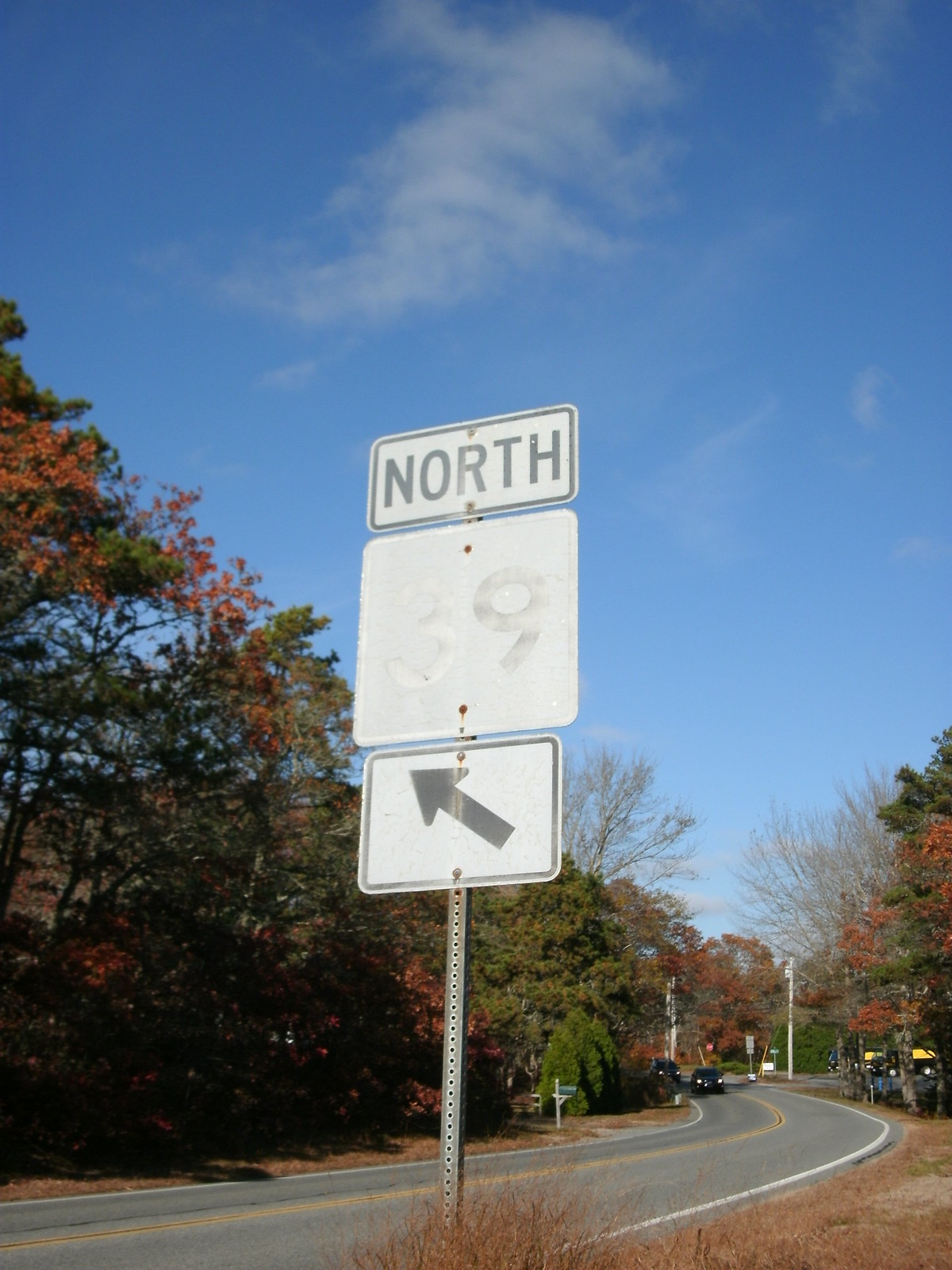This portrait-oriented image captures a faded street sign composed of three distinct parts mounted on a single metal pole. At the top, a horizontal rectangular sign reads "NORTH" in capital black letters on a white background, surrounded by a black border. Below it is a square sign, severely faded, that can be deciphered to read "39," although the numerals are barely visible. The bottom sign is another horizontal rectangle, featuring a black arrow pointing to the top left of the image, also set against a white background with a black border.

The setting reveals a curved road that enters from the bottom left and bends towards the center, then to the left. Two black cars are approaching from this curve. The road itself is divided by a solid double yellow line. Flanking the street are green and reddish autumn-hued trees, some with red flowers. The ground around the sign has a brown, fall-like tint. In the background, additional poles are faintly visible, adding depth to the scene. Above, a vibrant blue sky with sparse wispy white clouds crowns the composition.